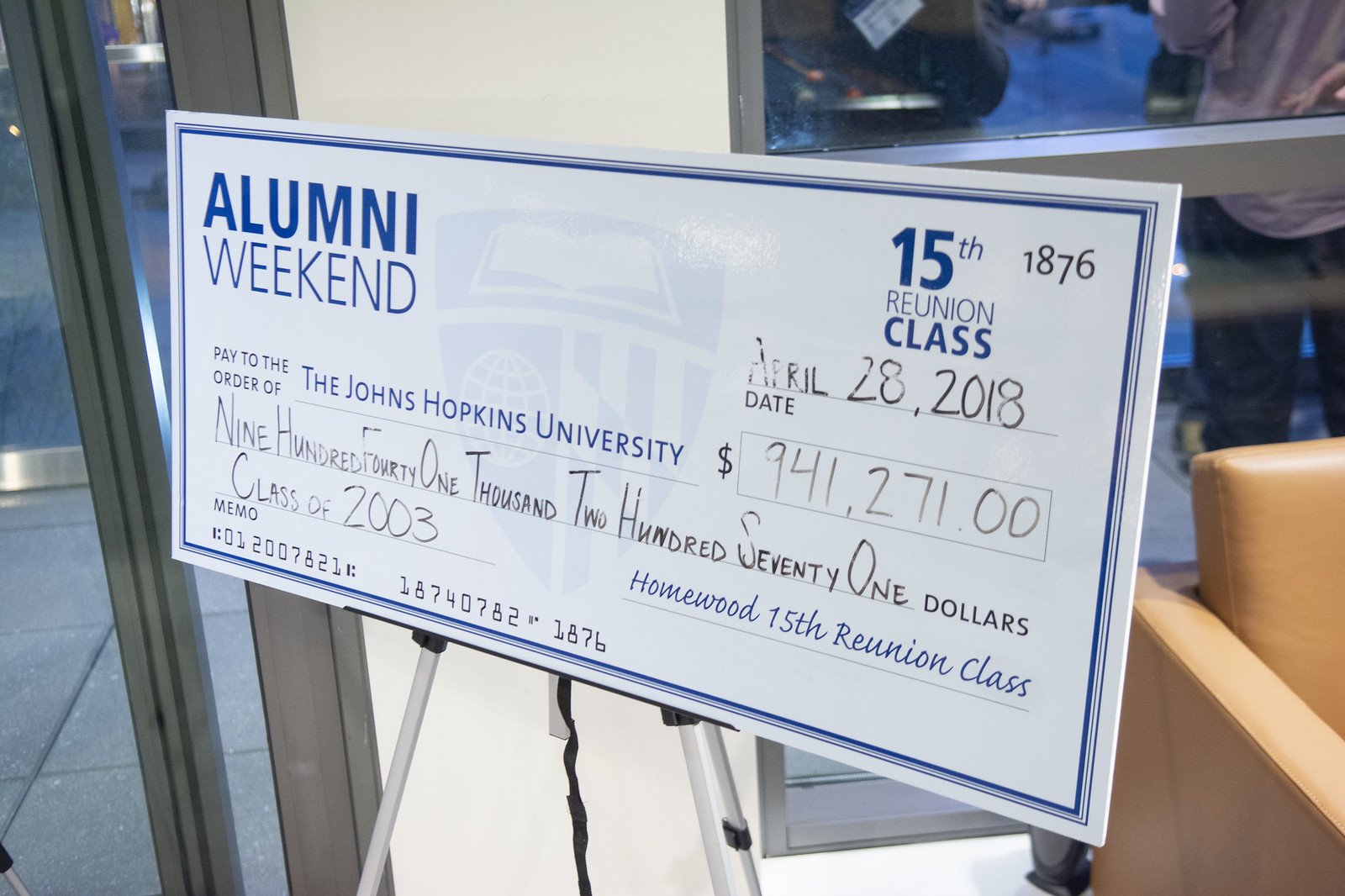This photograph captures an indoor event featuring a large oversized check placed at an angle, possibly on a counter, within an area that seems like a business setting. The check, designed to mimic an actual bank check, serves as a display for a generous donation. It has a white background with a narrow blue border and a lighter blue stripe. In the background, we can observe a beige or tan leather chair to the bottom right, and some seating with a tan-gold color. Through the glass windows behind the check, partial images of people can be seen, with some individuals notably wearing pinkish shirts paired with dark gray or black pants.

The check prominently features "alumni weekend" in bold blue text on the upper left corner, and "15th class reunion" on the upper right. The check number is 1876, and the date "April 28, 2018" is handwritten in black. The check is made out to "Johns Hopkins University" for the substantial sum of $941,271, which is both handwritten and displayed numerically below that line. The memo notes "class of 2003". The check is signed "Homewood 15th class reunion," including a routing number typically found on bank checks. This image effectively showcases the celebratory acknowledgment of the Class of 2003's significant contribution.